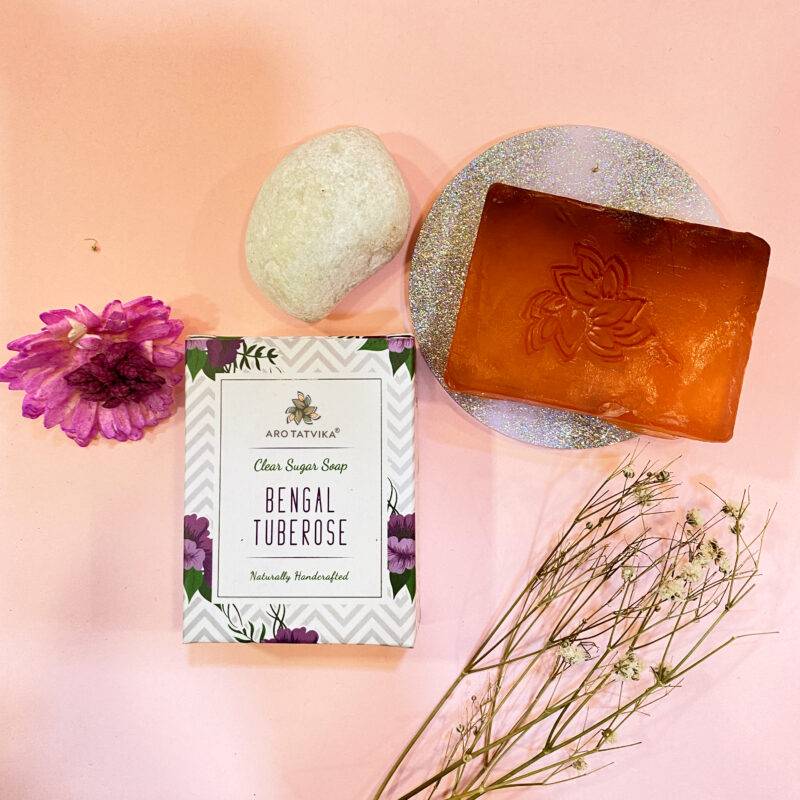The image features a collection of artfully arranged products set against a pink-peach background. At the top left sits a striking purple flower, its petals transitioning from light purple to darker hues towards the center. Adjacent to it is a light grayish-white, oval-shaped rock, and next to that, a circular dark gray disc with white dots, which likely serves as a soap dish. Positioned on this dish is a large, rectangular bar of soap, with a gradient of orange-brown to dark orange-brown, engraved with rose petal designs. 

In the bottom right corner, a sprig of dried flowers with green leaves and small white blossoms introduces a touch of natural elegance. Dominating the center of the image is a white rectangular package adorned with gray zigzag lines and purple floral motifs. The label reads "Arrow Tat Vika Clear Sugar Soap Bengal Tuberose Naturally Handcrafted." The soft pink background and the subtle shadows from the objects suggest gentle lighting from above, adding depth and warmth to the scene.